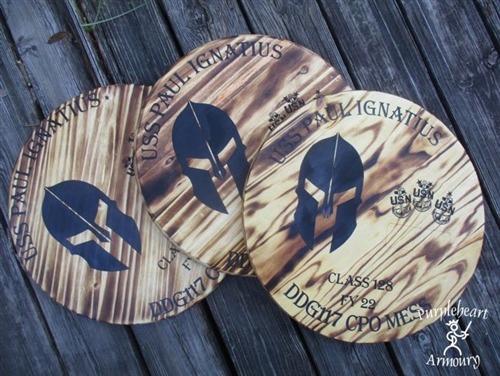The image is a full-color, square-shaped promotional photograph showcasing three round wooden tokens or coasters, arranged side by side with slight overlapping, the center one positioned slightly higher than the others. Each token prominently features a black illustration of a Spartan-style helmet with eye slits, a ridgeline, and face flaps. To the right of the helmet are three United States Navy seals. Encircling the top of each token is the text "USS Paul Ignatius," while the bottom reads "DDG 117 CPO Mess" with the identifier "Class 128 FY 22" above it. These wooden items, resembling coasters, appear to be designed by or for a naval context. They are made to look like wood, though it is unclear if the material is genuine or synthetic. The background consists of dark gray, weathered wooden slats, adding a rustic feel, and the bottom right corner bears a logo for "Purple Heart Armory," featuring a stick figure wielding a sword.